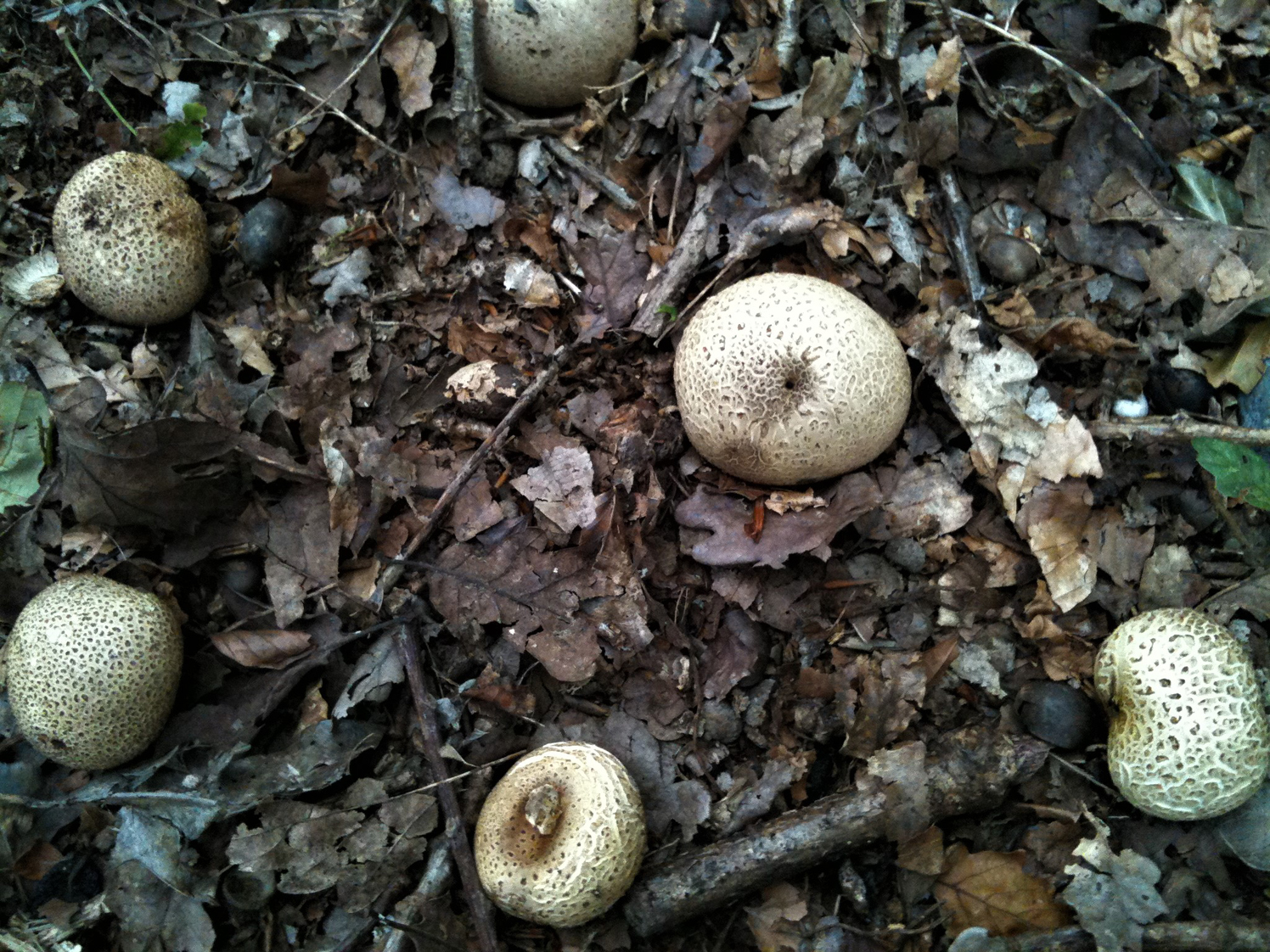In the aftermath of a rainstorm, six large mushrooms emerge from the damp forest floor, surrounded by wet leaves. Most of the mushrooms' stems remain hidden beneath the surface, except for one in the upper left corner which shows its stem clearly. These newly grown fungi resemble heavily roasted marshmallows with their textured caps. The diffused light from an overcast sky casts a muted glow across the scene, devoid of sharp shadows, enhancing the fresh, moist ambiance of the natural setting. Scattered smaller mushroom bits and leaves contribute to the rich, earthy composition of the image.